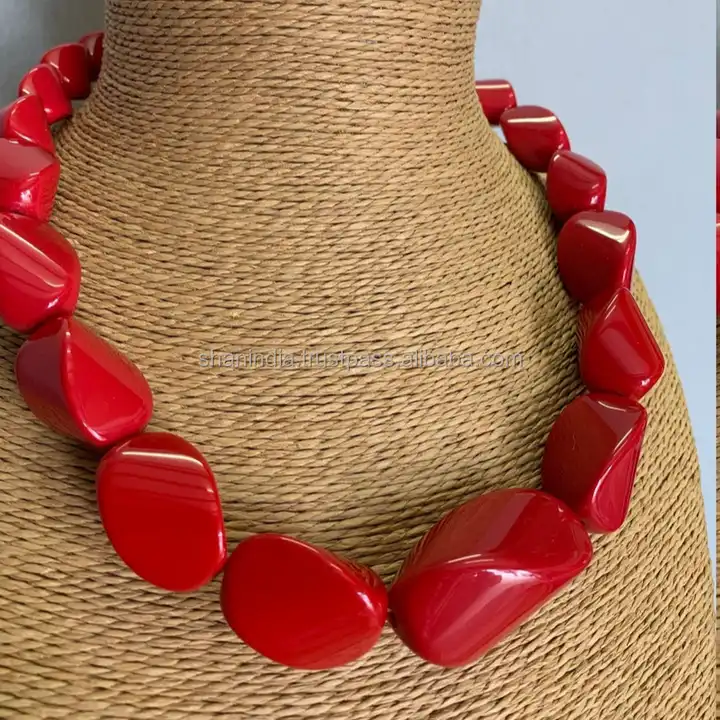This close-up photograph features a striking red necklace composed of large, chunky stones, each uniquely shaped and vividly bright. The necklace is relatively short, designed to sit snugly around the neck rather than hanging low. It is displayed on a mannequin-like form, which is actually a stiff, woven object made to resemble neck and shoulders, wrapped in very thin rope. The background of the image is light blue, although it's cropped tightly around the subject, rendering the setting indistinguishable. A subtle overlay, almost blending into the setup due to its light, almost invisible typography, reveals a website, possibly reading "Shanna Shanna India disperse family.com alabria.com," indicating that the image is sourced from a webpage. No clear branding or ownership details are provided for the necklace in the image.